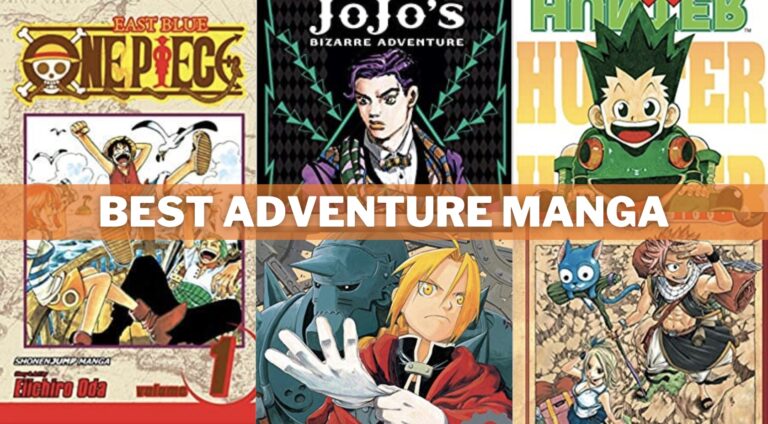This vibrant color image features a compilation of three distinct manga covers, each portraying dynamic and detailed cartoon drawings, under a translucent brown banner with white, all-capital letters declaring "BEST ADVENTURE MANGA". 

On the left, the cover for "East Blue One Piece" showcases a lively scene with a skull and crossbones forming the "O" in "One". A kid in a red tank top and blue shorts is depicted with one arm bent, a leg kicked up, and his mouth wide open, possibly yelling. He's on a boat surrounded by white clouds and seagulls, indicative of an ocean-bound adventure. Several other characters and elements, including a figure with red boots and a bug head with googly eyes, add to the dynamic battle scene happening on the boat, highlighted by its yellow background and red-bordered details.

In the middle, the cover of "JoJo's Bizarre Adventure" features a striking contrast between two characters. At the top, a man with neatly combed, purplish-black hair, wearing a purple suit jacket and multiple colorful scarves, gazes off to the left with a mixed look of shock and determination. Below the title banner, another character with shaggy blonde hair, dressed in a popped-collar black cloak lined in white as well as a red cape, prepares to don white gloves. A large, teal, horned monster looms behind him, adding an element of otherworldly intrigue to the scene.

The rightmost cover, likely of "Hunter x Hunter", depicts a young, cheerful boy riding a giant frog, his wide smile and energetic pose capturing a sense of joy and adventure. A background character, possibly a blue cat with bugging eyes, and additional figures including a genie-like humanoid with a mischievous grin and a buxom woman, contribute to the whimsical and fantastical atmosphere of the scene, adorned with vivid colors and intricate character designs punctuated by orange and yellow title elements.

Combining these elements, the detailed compilation gives the viewer a spirited glimpse into the thrilling and diverse worlds of adventure manga.